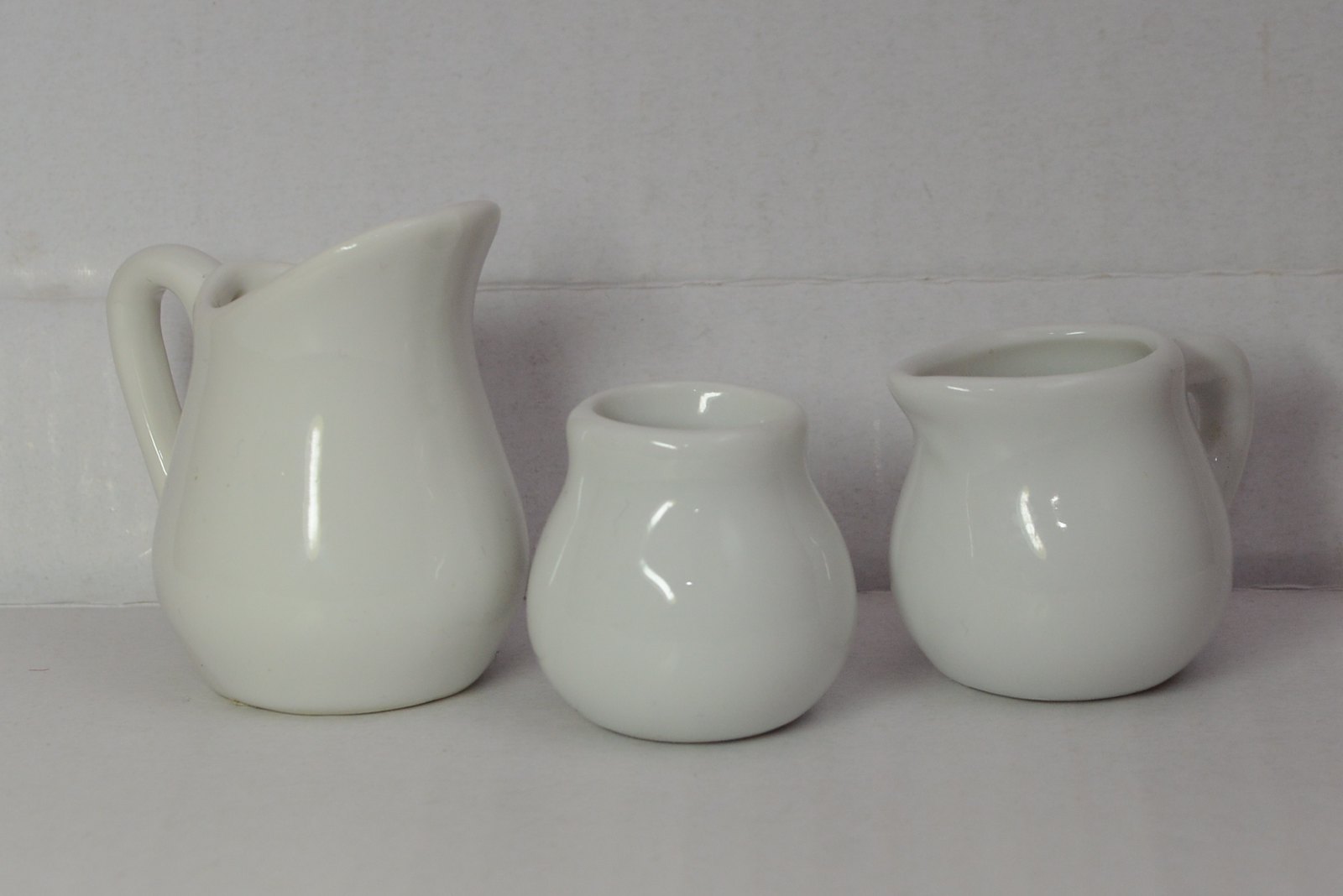In this color photograph, a bright white scene is set against a white brick background and a pristine white tabletop. Center stage are three glossy white ceramic pitchers. On the left stands the tallest pitcher, distinguished by its elongated, curved spout and reminiscent of a classic iced tea pitcher. Front and center is a shorter, squat ceramic container with a wide base and circular top, perfectly suited for holding sugar or similar contents. To the right, a medium-sized pitcher, slightly shorter than the tallest one, features a prominent handle aligned to the left and an angled spout, making it an ideal creamer jar. Each pitcher’s ceramic finish gleams under the light, creating a harmonious and visually striking arrangement.